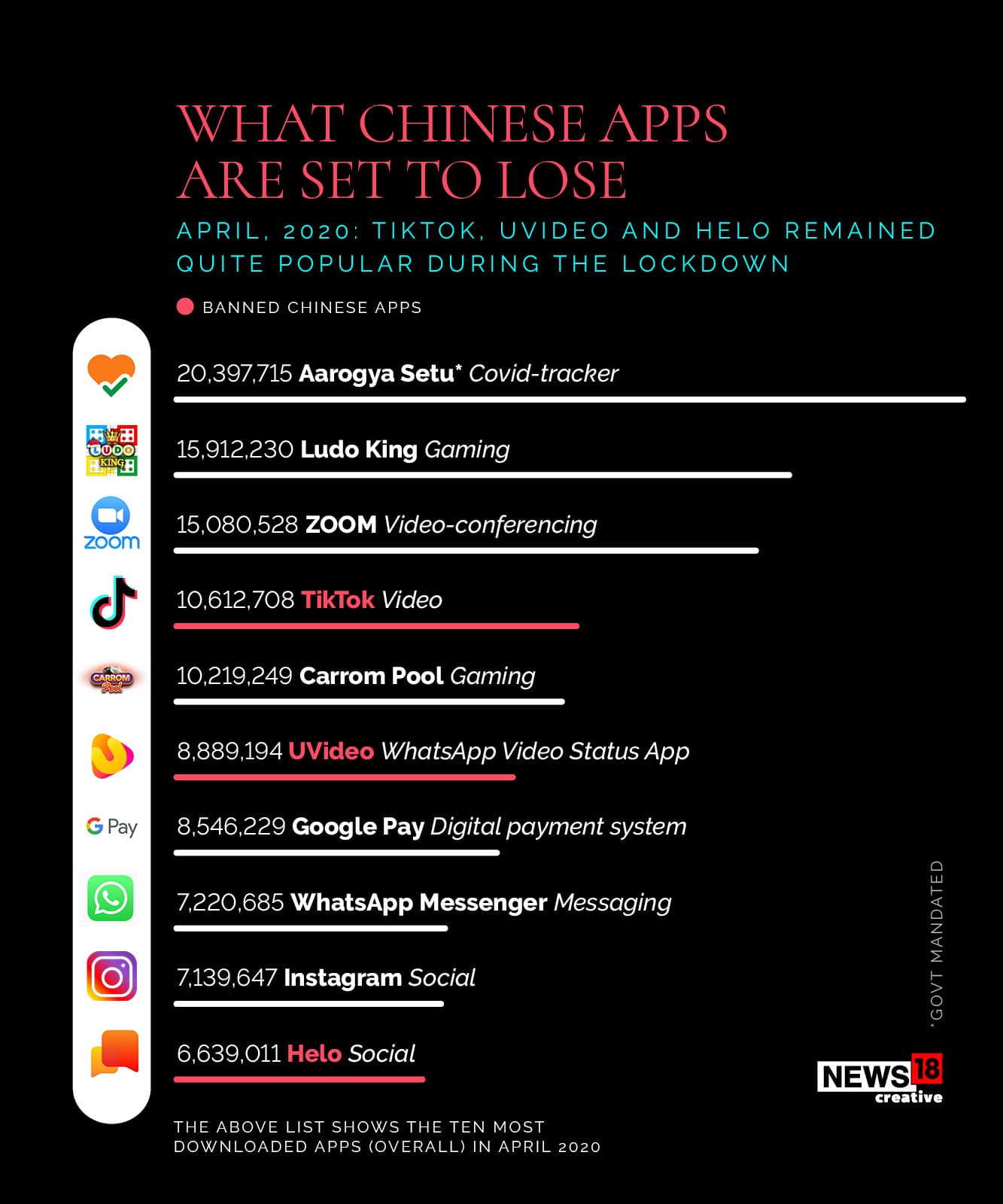**Infographic Analysis: Impact on Popular Chinese Apps**

The infographic, set against a sleek black background, provides a detailed examination of the shifting landscape of app usage amid the April 2020 lockdown. At the forefront, in bold salmon pink text, the headline reads: "What Chinese Apps Are Set to Lose." Beneath this, in subdued greenish-blue text, is the context: "April 2020: TikTok, YouVideo, and Hilo remained quite popular during the lockdown."

Significantly, a highlighted pink dot indicates the "Banned Chinese Apps." The apps listed in pink—TikTok, YouVideo, and Hilo—represent these banned applications. The infographic then transitions into a comprehensive bar chart detailing the download figures of various apps in descending order.

Atop the chart is Aarogya Setu, a COVID-19 tracker app, leading with an impressive 20,397,715 downloads. Following is Ludo King, a gaming app, with nearly 16 million downloads. The Zoom video conferencing app occupies the subsequent position, trailed by TikTok (marked in pink to denote its banned status).

The list continues with Karam Pool, another gaming app, followed by YouVideo (also in pink), WhatsApp, Status Video, Google Pay, the WhatsApp Messenger, Instagram, and finally, Hilo (marked in pink) which recorded almost 7 million downloads. This detailed snapshot presents a clear view of app popularity and the impending loss faced by the banned Chinese apps, emphasizing the shifting digital landscape amid regulatory changes.